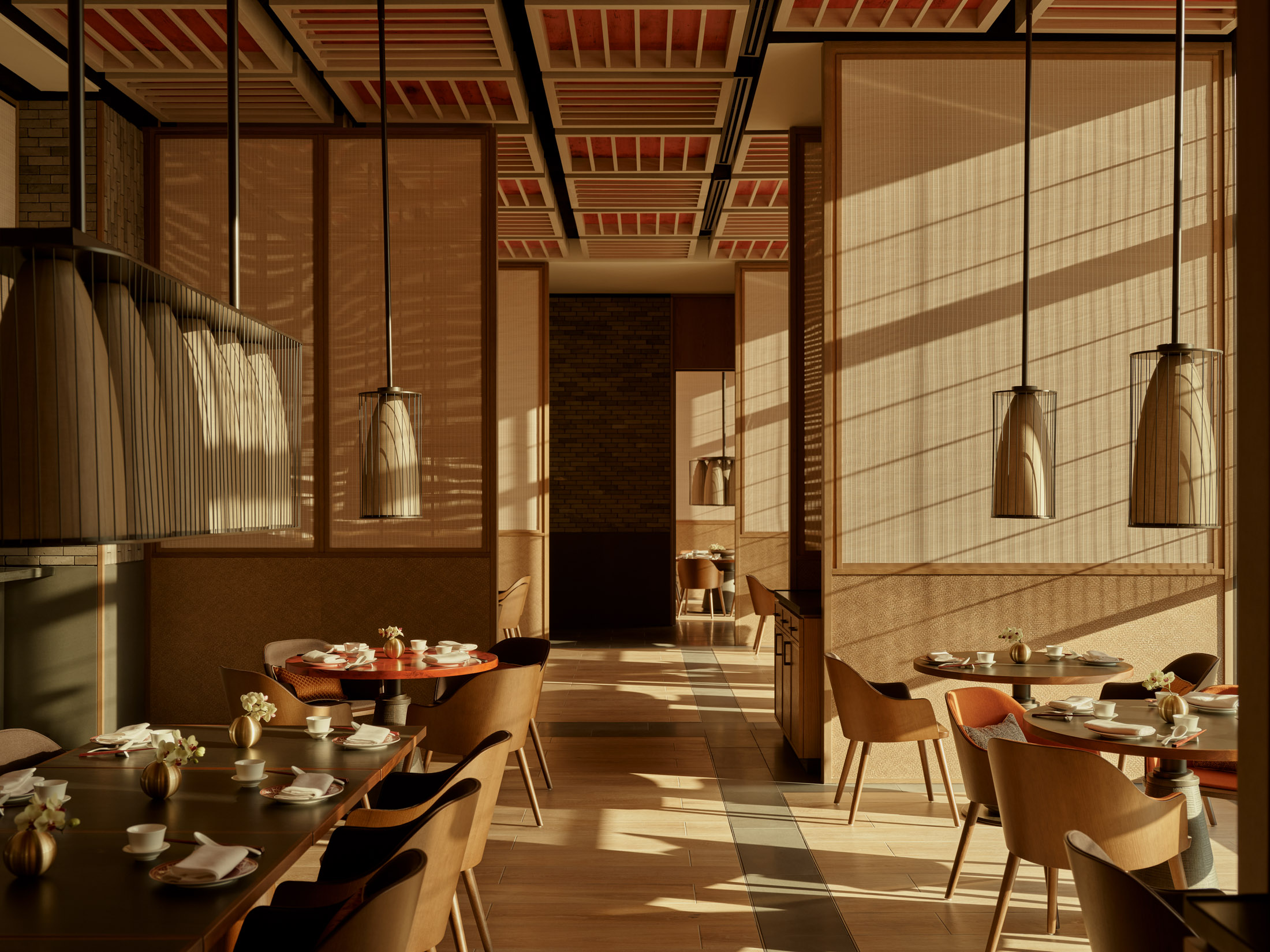This image showcases the interior of a high-end, modern restaurant infused with Japanese design elements. The space features tan and brown walls, with partition walls resembling traditional paper windows framed by wood. The lower portion of the walls and the ceiling follow a tan color scheme, while the back wall is a mix of brown and tan bricks with a darker brown base. The seating area includes mid-century chairs with dark brown seats and lighter brown sides, paired with circular and rectangular tables that have dark brown tops and lighter brown sides, supported by black legs. Unique to the décor, some tables sport a round red top. The tables are set with plates, napkins, knives, and teacups on saucers, ready for service. Modern-day lanterns and pendant lights with cage designs hang from black poles, providing an elegant lighting solution. The floor design consists of green lines contrasting with brown wood. The space appears to be well-lit with the sunlight streaming through the windows, adding warmth to the overall tan-dominated color palette.